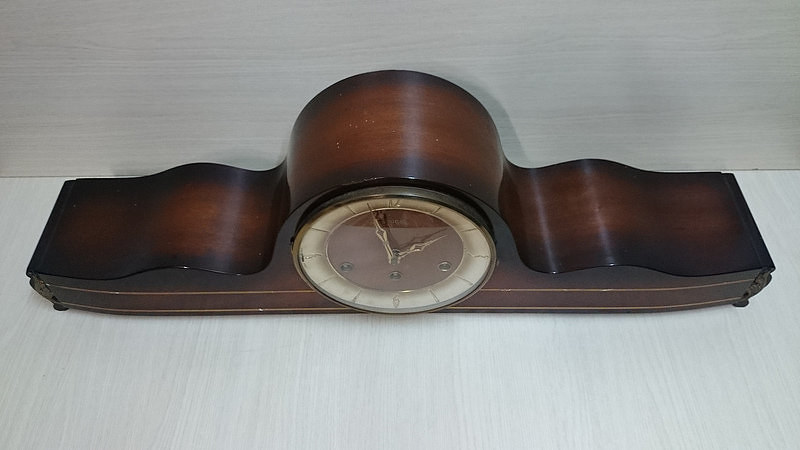The image depicts an ornate, antique wooden mantel clock resting on a white laminated surface with faint vertical grey stripes, seamlessly blending into a similarly laminated wall boasting a horizontal light grey woodgrain pattern. The clock, crafted from dark-stained wood, features a distinctive round face encased in glass, allowing for its winding via three visible keyholes. The ivory-colored clock face showcases gold hands indicating it is just before two o'clock, with numbers at the 12, 3, 6, and 9 positions and simple lines marking the remaining hours on a whitish border. The central part of the face, where the hands are anchored, is also wooden. The clock extends horizontally, presenting an undulating, wave-like pattern on either side of the round center, reminiscent of a signature piece suitable for prominent display on a mantel, large desk, or chest of drawers.